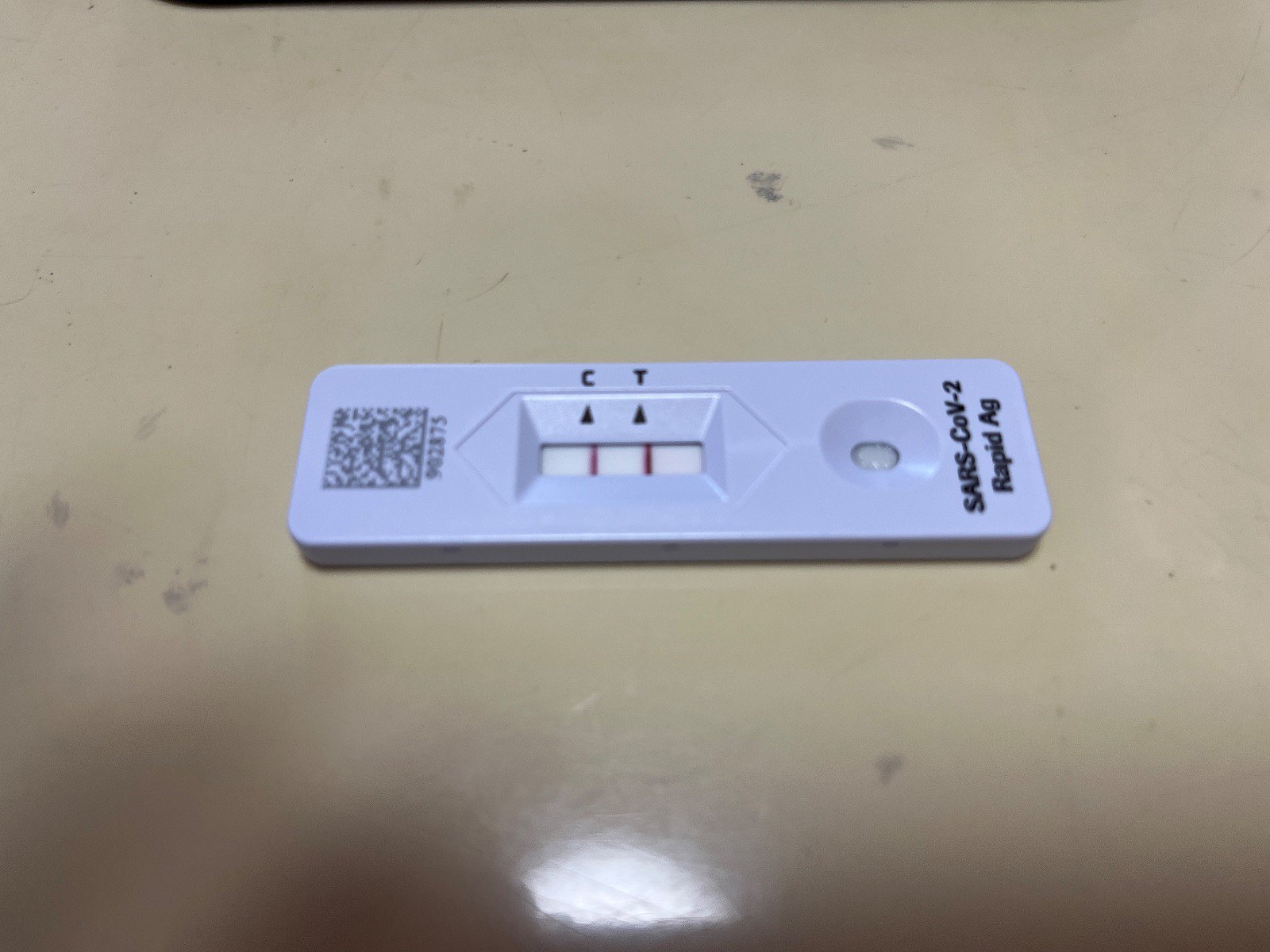In this photograph, a COVID-19 rapid antigen test is prominently featured against a visibly dirty beige countertop. The surface of the counter is marred with numerous scuffs, scratches, and even black marks near the top middle. Faint pencil lines are also discernible among the imperfections. A bright fluorescent light casts an intense glow over the scene, highlighting the overall grime and creating shadows that may delineate the outline of a hand or arm. The COVID-19 test itself has a UPC mark at the top, labeled "902875." The test is clearly marked "SARS-CoV-2 Rapid Antigen Test (AG)" and features an oval opening designed for applying drops of testing fluid. The indicator area displays two vivid red lines next to the letters "C" and "T," signifying a positive result for COVID-19. The red lines are strikingly intense, resembling a deep, almost blood-red hue.